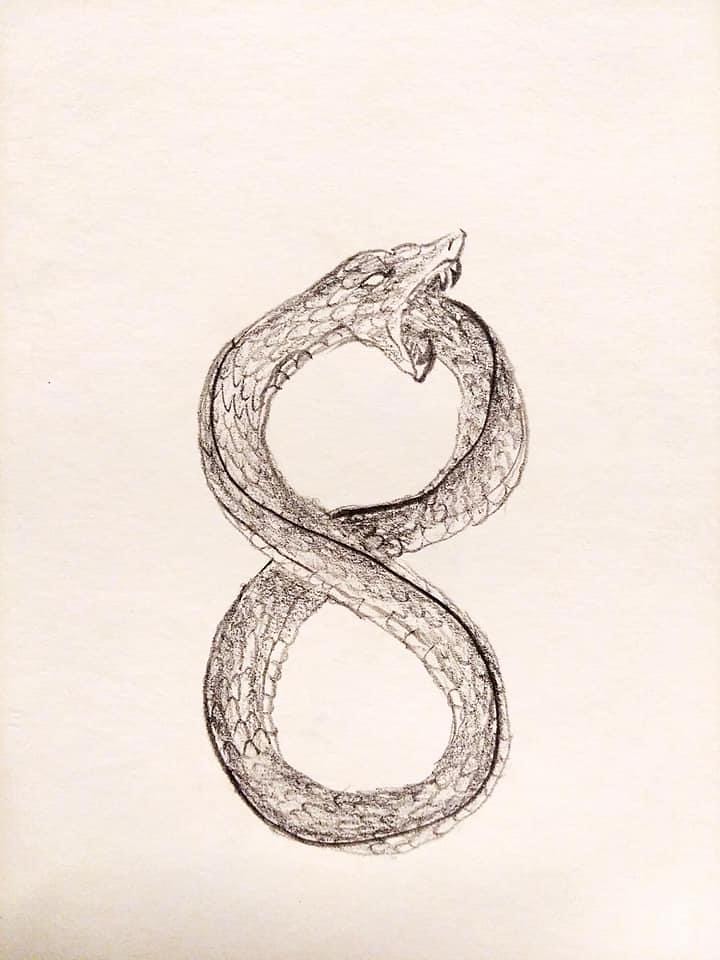This is a detailed drawing of a snake, evocatively rendered on cream-colored paper. The snake, inked primarily in grayish-black hues with some brown tones, forms the silhouette of an infinity symbol or the number 8 by wrapping its body in a continuous loop. The drawing captures the nuanced textures of the snake's scales, and its sinister demeanor is accentuated by intricate features such as a pointed nose, glaring white eye, and visible fangs. The head of the snake, positioned at the top of the figure, is depicted with an open mouth that bites its own tail, embodying the ancient symbol of the Ouroboros. The light brown-gray background enhances the starkness of the snake, and there are no additional texts or elements, drawing the viewer's focus solely to this striking, symbolic illustration.